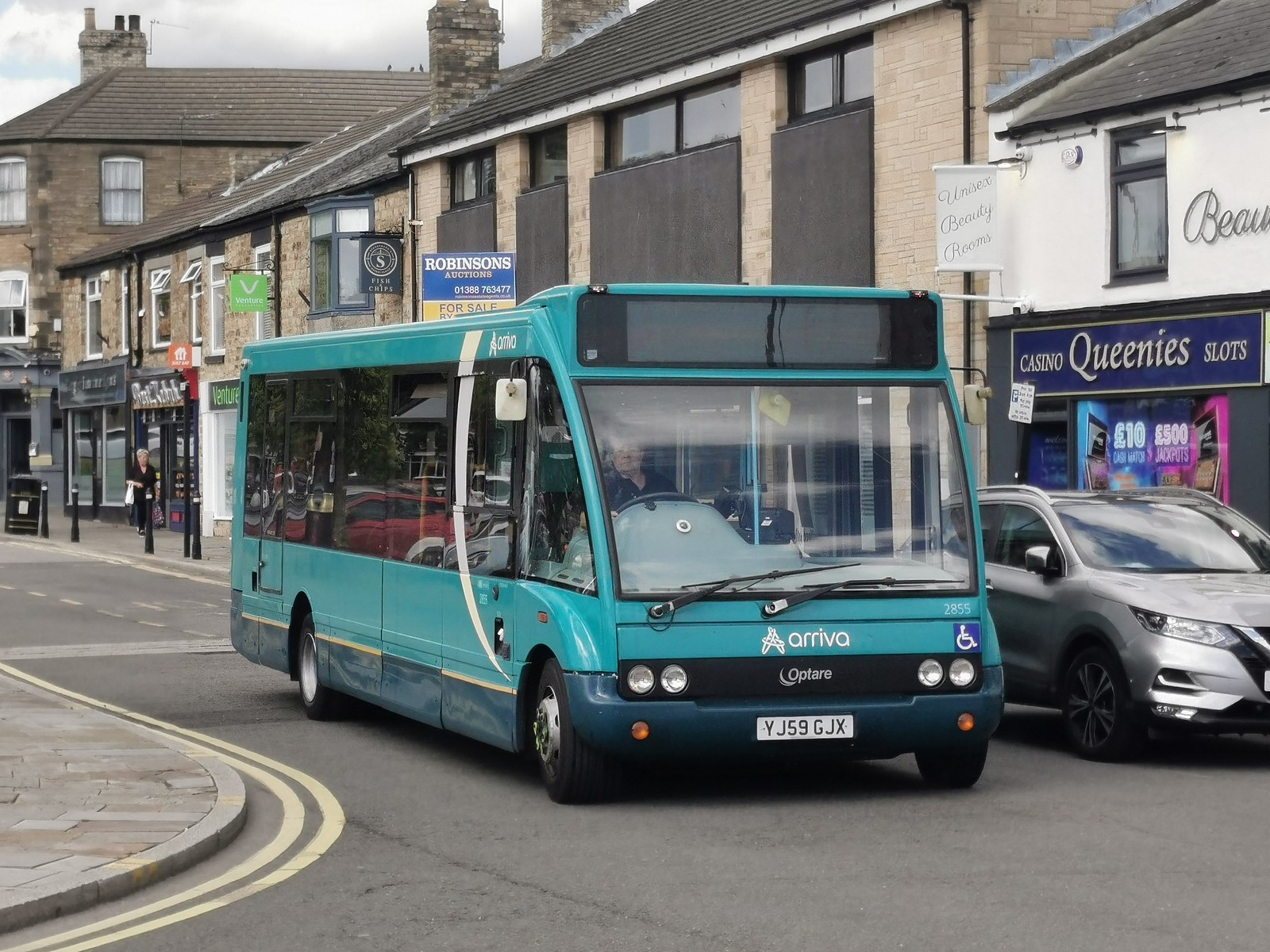This photograph captures a small shuttle bus and a silver car on a town street. The bus, identified as an Arriva Optair with license plate YJ59GJX, features a greenish-blue (cyan) color scheme with a darker navy blue bottom portion and a yellow stripe alongside it. The bus number 2855 is printed on the green front bumper along with a handicap sign below it. The driver, an older gentleman in a navy blue outfit, has his hands on the steering wheel. The bus's digital sign is currently off. Positioned near the bus is a new, silver car. Both vehicles are located on a small city street bordered by two-story buildings housing various shops, including Venture, Fish and Chips, Robinson's Auctions, Unisex Beauty Rooms, and Casino Queenie's Slots.